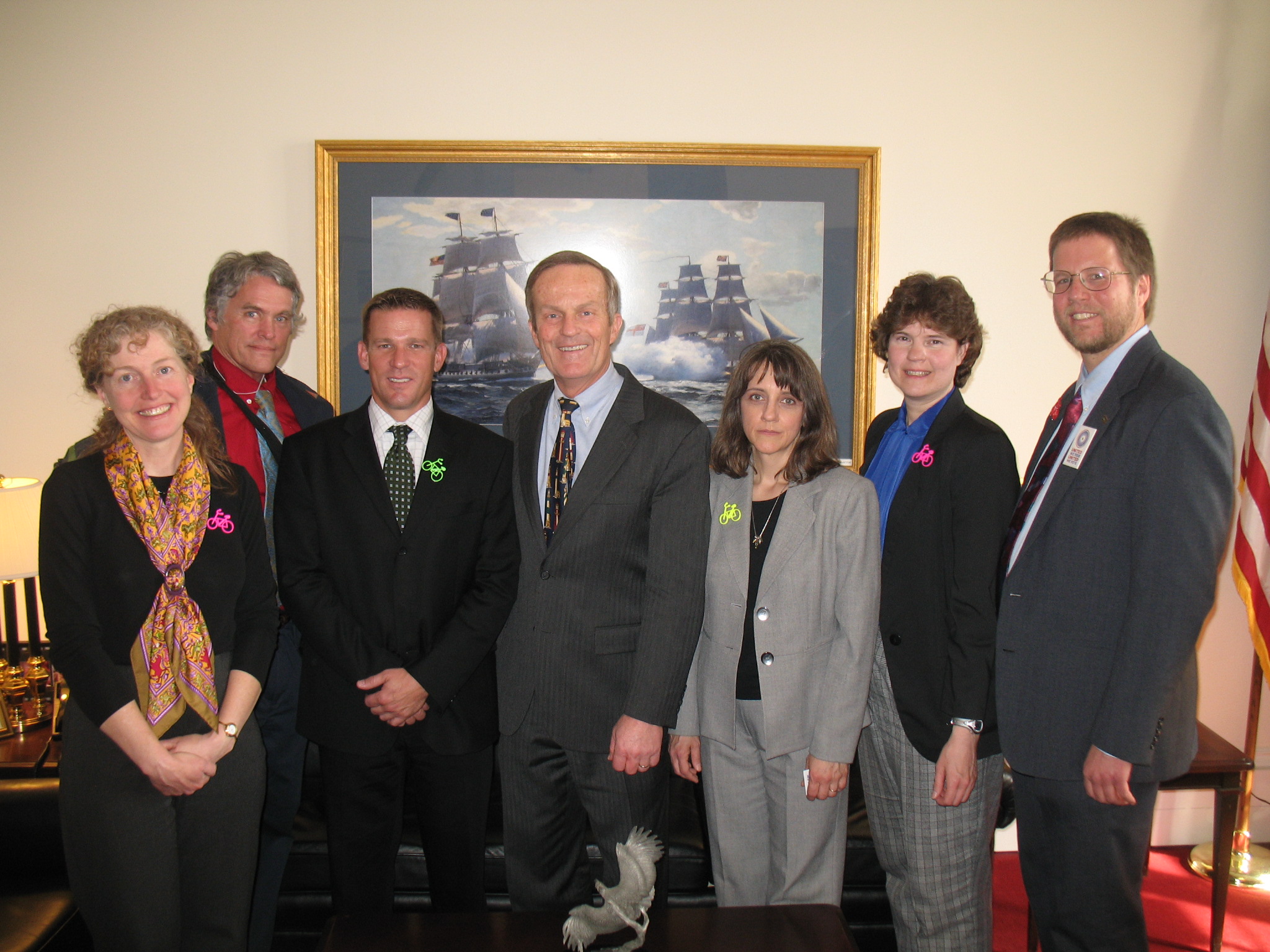In this color photograph, a group of eight individuals, comprising both men and women, are posing in a formal setting. Each is dressed in business attire, with the men in suits and the women in pantsuits, standing on a red carpeted floor. The backdrop is stark white, adorned prominently with a large, gold-framed portrait depicting two sailing ships engaged in battle, evident by the billowing clouds of smoke and cannon fire. To the right of the group stands an American flag on a pole, while off to the left, a table with a lamp is visible. Behind the group, there’s a mix of fine brown tables and a black leather sofa.

From left to right, the first individual is an older woman in a black top, accented by a yellow and purple scarf tied around her neck. She wears a distinct pink bicycle pin on her chest. Behind her, a man with gray hair sports a blue and red jacket with a strap across his body. Next is a young man with light brown hair and fair skin, wearing a black suit and a green and white checkered tie, and he also has a green bicycle pin.

In the center stands an older man in a somewhat textured black suit, white shirt, and patterned black tie, smiling warmly. To his right, a woman in a gray suit and black top appears less enthused, possibly tired. She has brown hair, a necklace, and a yellow bicycle pin on the opposite side from the others. Beside her, another woman with curly brown hair dons a black suit jacket, a blue blouse, and checkered gray pants. Her pink bicycle pin contrasts with the others. Finally, the last person on the right is a man with short brown hair, a light beard, and glasses. He wears a gray suit with a red tie and has a white card pinned to his lapel.